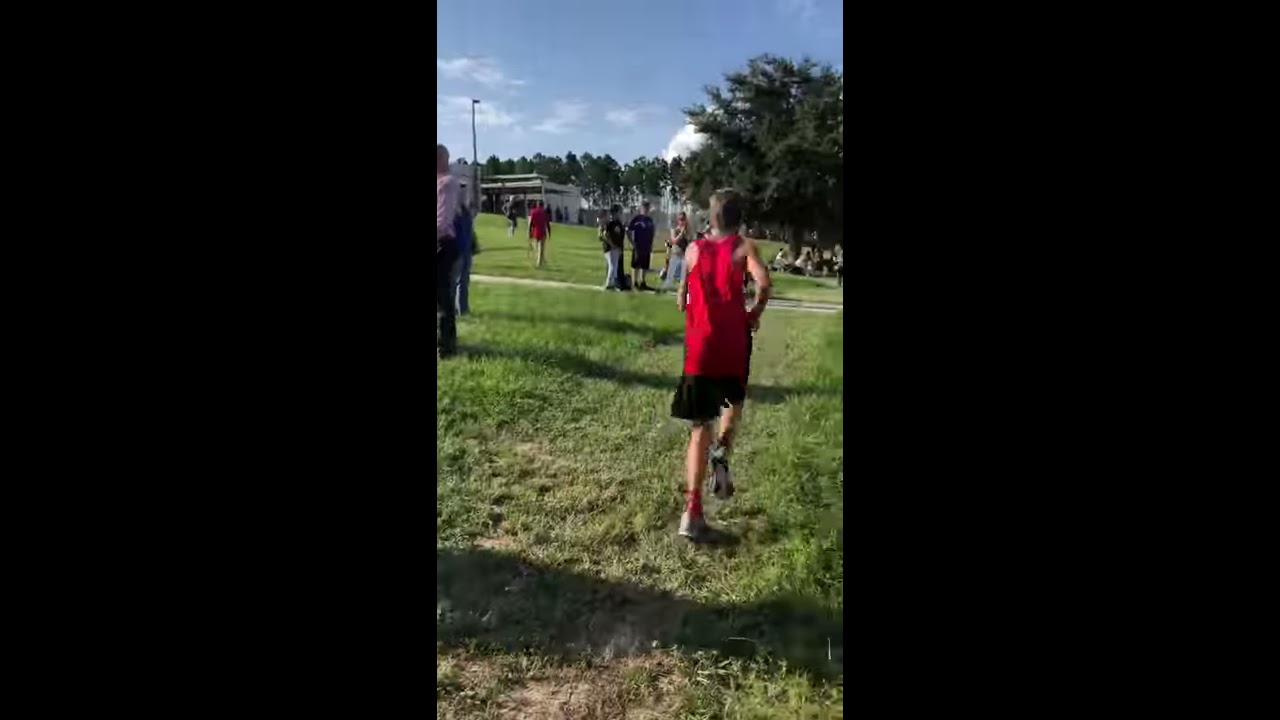The image is a vertically framed photograph with thick black bars bordering the left and right sides. It captures a vibrant outdoor scene in a park during the daytime. The central focus is a boy or young man, likely of Caucasian descent, caught mid-stride as he runs away from the camera. He has short brown hair and is attired in a red tank top that flows untucked over his black shorts, complemented by white sneakers. The path he runs on curves to the right and is part of a mowed grassy field that stretches from the bottom to the center of the image. Scattered throughout the park are people in various groups, some standing, others sitting beneath trees in the distance. The backdrop of the photograph features a horizon with a white office building and a tall light pole, partially obscured by abundant green trees. The sky above is a soft periwinkle blue, dotted with scattered clouds, enhancing the overall daytime ambiance of the scene.